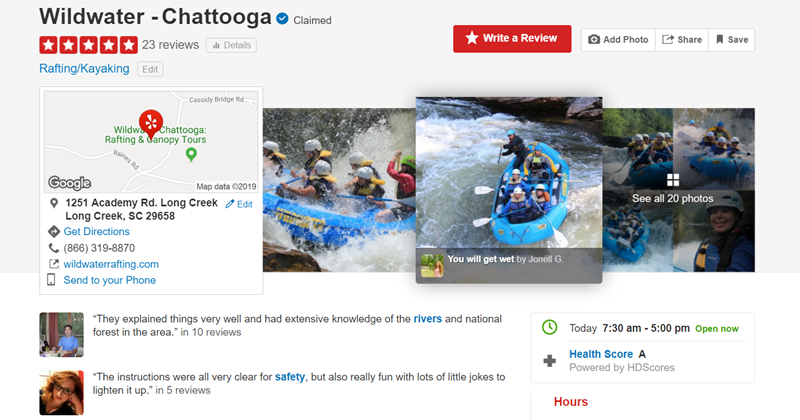This rectangular image, oriented horizontally, appears to be either a Yelp ad or a Google review ad for "Wildwater-Chattooga," a rafting and kayaking service. The top section of the image features a gray box containing the business name "Wildwater-Chattooga," along with its rating of five stars, based on 23 reviews. In the upper left corner, navigation options are available, including "Write a review," "Add photo," "Share," and "Save."

Directly below this, contact information is prominently displayed, including a map, address, email, phone number, and options like "Get Directions" and "Send to your phone." To the right side, there are three thumbnail images showing people rafting on a river with options to view additional photos.

The bottom section of the image showcases a few customer reviews. One review praises the detailed explanations and extensive knowledge of the local rivers and national forests provided by the staff. Another review commends the clear safety instructions and mentions that the experience was made fun with lighthearted jokes. In the bottom right corner, operational details are noted, including business hours (open from 7:30 a.m. to 5 p.m.) and a health score of 'A.' However, the section labeled "Hours" has no further details listed.